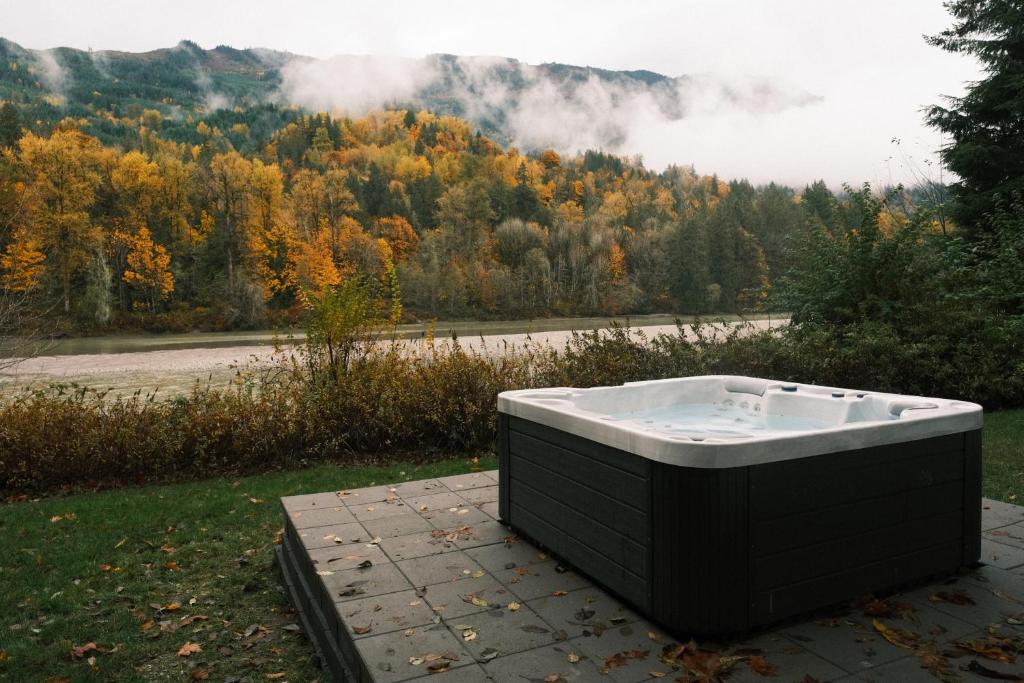In this serene landscape image, the foreground features a black and white, square-shaped hot tub with black wood siding set upon a tiled platform. The inside of the hot tub is white, with water visible inside. The platform consists of several square tiles, around which lies a grassy yard dotted with golden-yellow leaves, likely fallen from the surrounding trees hinting at the autumn season. To the side of the hot tub, you can see a pine tree and nearby bushes. As you gaze beyond, there is a river or lake bordered by a wall of bushes separating the hot tub area from the expansive forest in the background. The dense forest climbs up a hill, displaying a rich tapestry of greens and yellows amidst the changing foliage of fall. Higher up, the scene transitions to a mountain with wisp-like clouds or perhaps light fog partially veiling its peak and adding to the tranquil atmosphere. The image captures a seamless blend of natural beauty and human comfort, with no signs of civilization breaking the continuity of the serene, untouched wilderness.